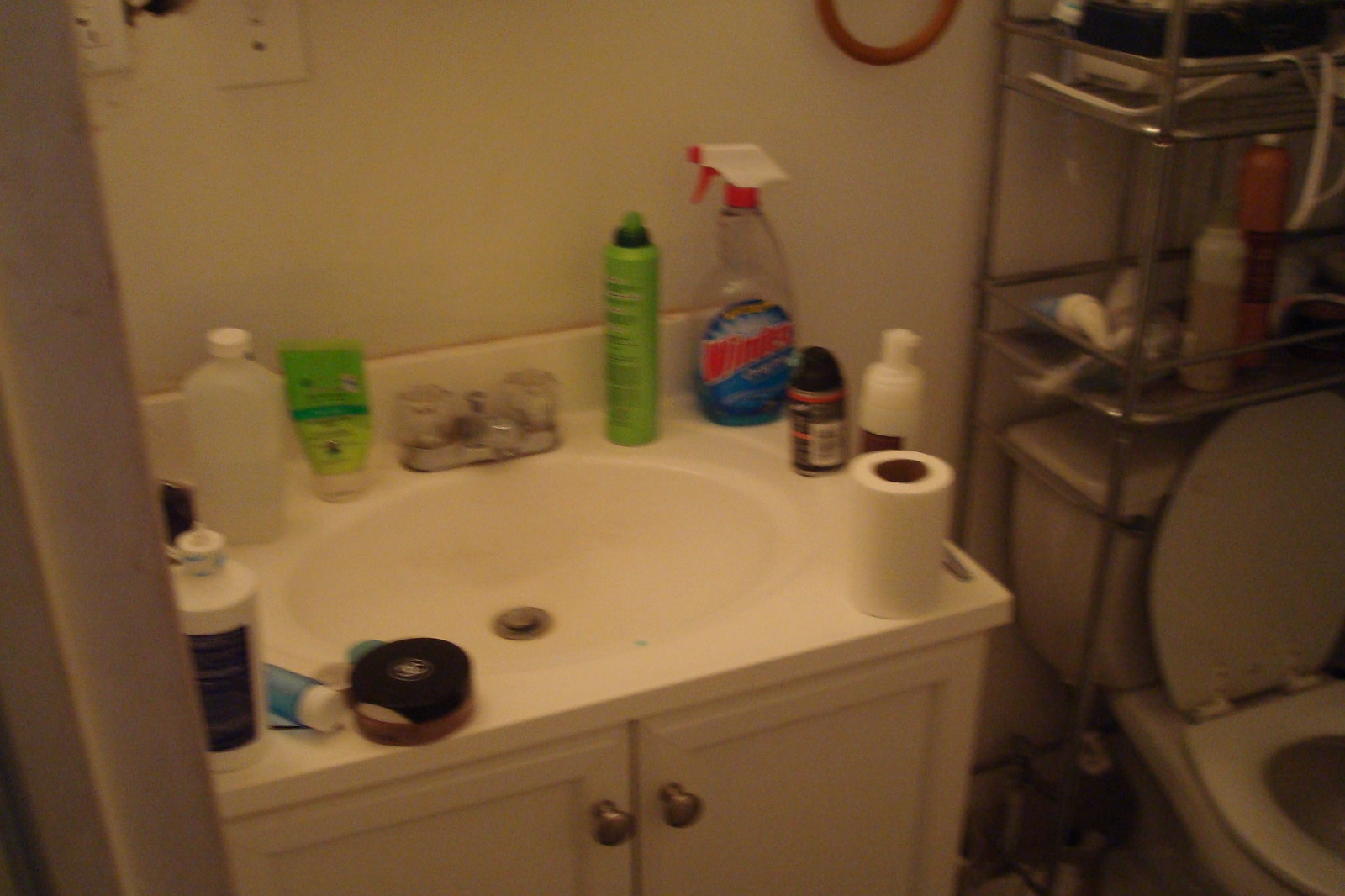The image depicts a rather cluttered and untidy bathroom. The walls are white, though somewhat dirty, featuring two electrical outlets. A small, rectangular white vanity with clear handle knobs for the faucet sits against the wall. The vanity's surface is cluttered with various items, including a toilet paper roll, a bottle of Windex, a can of hairspray, and other assorted supplies. Below the vanity, there are two white cabinet doors with silver knobs. To the right of the vanity is a white toilet with the lid raised. Above the toilet, a metal wire rack shelving unit is mounted on the wall, heavily laden with various indistinguishable items, adding to the sense of disorder in the room.